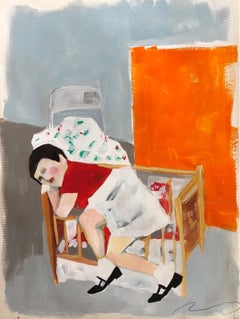The painting portrays a young girl with a lighter skin complexion, depicted in an abstract and modern style. She has short, black hair and is dressed in a red shirt paired with a white skirt. Her footwear consists of black shoes and white socks. The girl appears to be in a reclining or napping position on a crib-like object or couch, with a white blanket or possibly a pillow behind her head. The background of the painting features a solid orange rectangle, presumably a door, and a gray area representing a wall. The artwork is likely oil on canvas and presents an unusual perspective, characteristic of modern abstract art. The setting is brightly lit, bringing clarity to the composition's details.